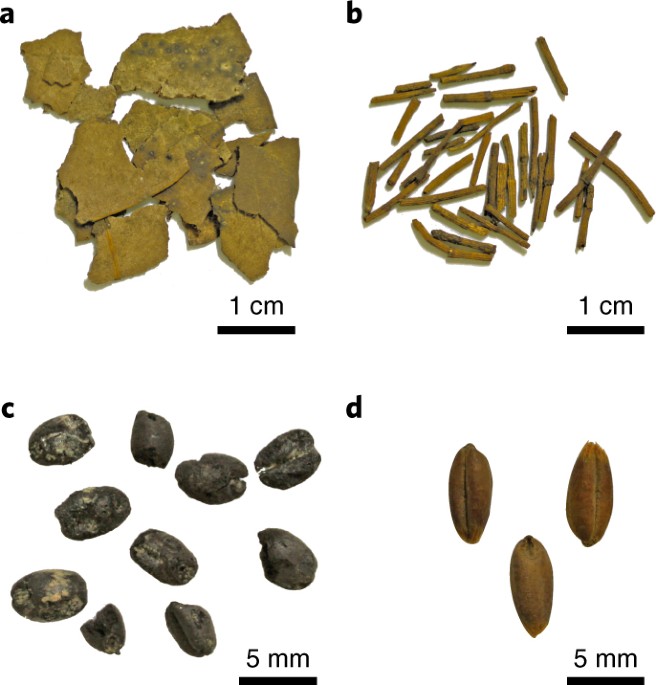The image displays four distinct natural items labeled A to D, with a white background and size scales indicated underneath each section. Item A, situated in the top left, consists of thin, flaky, goldish-brown sheets resembling either dried leaves or thin rock formations, marked as one centimeter for scale. Item B, found in the upper right, appears to be brown, leafless plant stems, similarly marked as one centimeter. Item C, located on the lower left, features dark, almost black seeds with occasional tan dusting, shaped like small ovals, with a five-millimeter scale. Finally, Item D, in the lower right, comprises elongated, oval-shaped nuts or seeds, brown in color and resembling pecans, also measured with a five-millimeter scale.